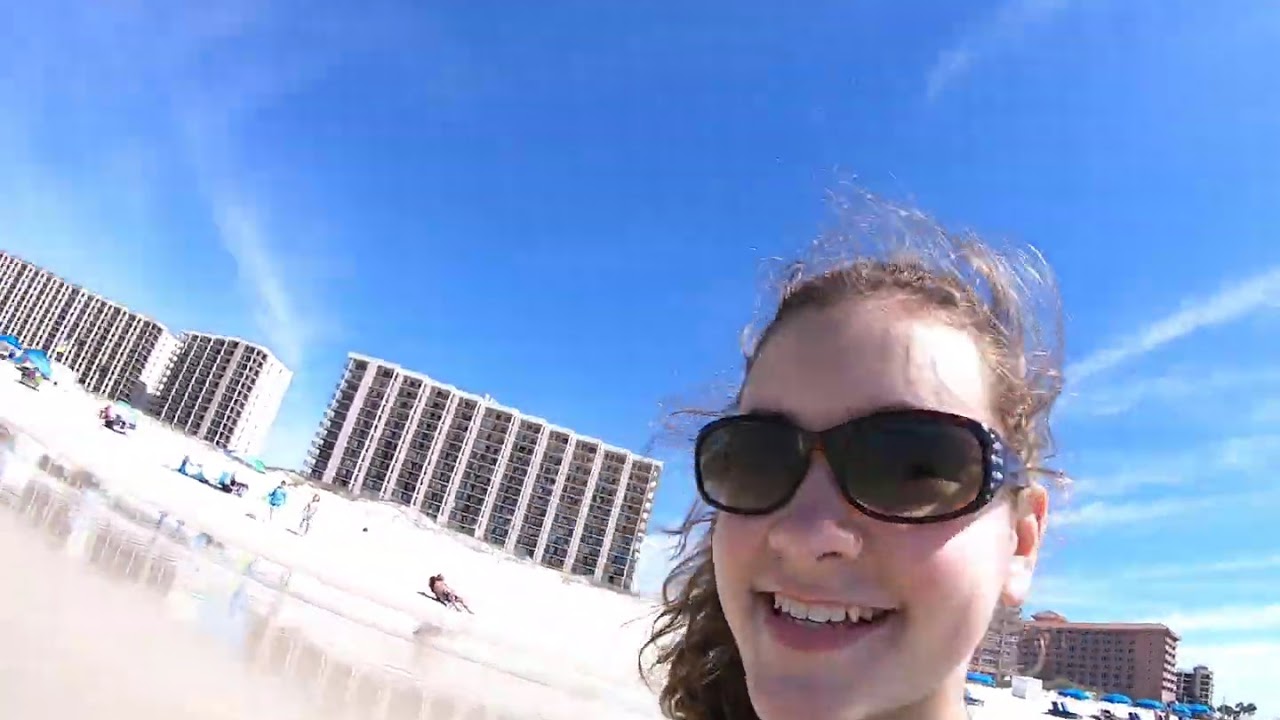The photograph captures a lively beach scene, seemingly taken outdoors and possibly a screenshot from a video due to noticeable compression. Central to the image is a close-up of a young girl, likely in her late teens or early twenties, with brown hair being playfully tousled by the wind. Her prominent, open-mouth smile reveals her upper teeth, and she is adorned with dark sunglasses embellished with rhinestones near the ears. The backdrop features a bustling beach flanked by rows of blue umbrellas and sunbathers sprawled across the white sand. The sandy area near the lower left corner appears wet, suggesting proximity to the shoreline. Beyond the beach, an array of towering hotels ranging from six to twelve stories high dominates the horizon, their white façades contrasting sharply against the vivid blue sky dotted with occasional clouds. The scene exudes a vibrant, relaxed atmosphere, reflecting a quintessential beach day likely at a resort.